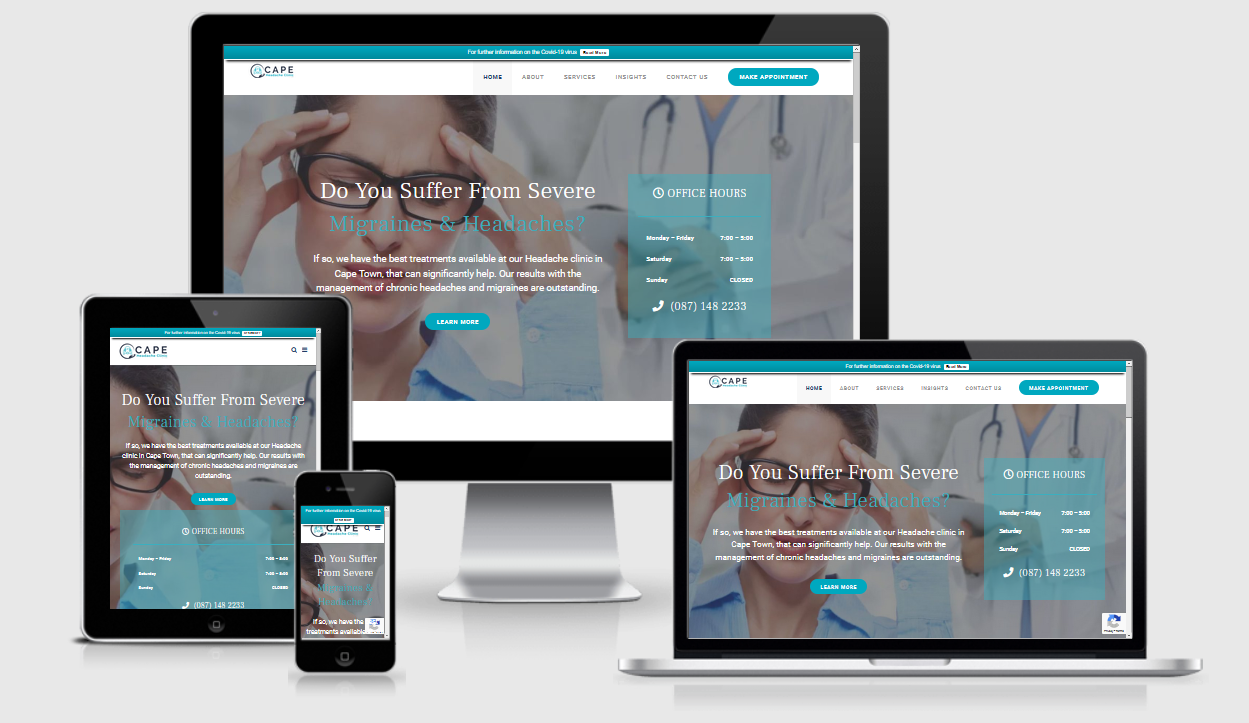The image features a meticulously organized setup of multiple electronic devices, each displaying the same webpage. The devices include a large computer monitor, a laptop, a tablet (possibly an iPad), and a smartphone, all arranged neatly against a light gray background. 

On each screen, there is a photo of a white woman, likely in her early 30s, wearing black-framed glasses. She appears distressed, with a frown on her face and her hands pressed against her temples. Superimposed on her photo is a headline in white and blue font that reads, "Do you suffer from severe migraines and headaches?"

Beneath this headline, there is smaller white text, unreadable due to its size. On the right side of the headline, a light sky-blue vertical rectangle contains the words "Office Hours" in white font, listing the working hours and a contact phone number at the bottom.

Additionally, on the left side of the image, there is a partial view of a doctor's figure, identifiable by the white coat and a stethoscope draped around the shoulders. 

At the very top of the webpage, there is a header that appears white with some black text on the left, likely spelling "CAPE" in capital letters. Next to this text is a circular logo, black with an indiscernible design. The top border of the webpage is a greenish-blue color, featuring a menu with several items that are too small to read.

Each screen shows the same website, appropriately formatted for the respective device type, enhancing the visual appeal and functionality across different platforms.